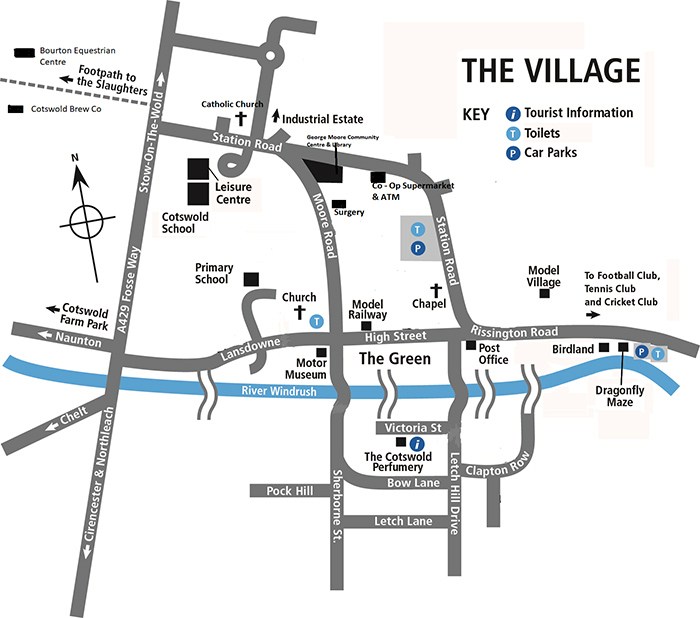This image is a detailed map of a neighborhood commonly found in a brochure or tourist pamphlet, displayed against a white background. In the upper right corner, large black letters read "The Village," and directly below, a key explains the various symbols. A dark blue circle with a white "I" indicates tourist information, a light blue circle with a white "T" signifies toilets, and a dark blue circle with a white "P" denotes car parks. The map features a gray-colored street layout with street names in white text. Prominent roads include High Street, Rissington Road, Lansdowne, Naughton, Cerencester, North Leach, A429 Fossey Way, Stowe on the Wold, and Station Road.

A horizontally flowing river named River Windrush crosses the center of the map, with four bridges indicated at various points. Key landmarks are marked using different symbols: small black squares for buildings, “X” for churches and chapels, and square boxes for educational institutions like the Cotswold School and a primary school. Additional points of interest include a Catholic Church, the Green, a Motor Museum, a model railway, a post office, Birdland, and the Dragonfly Maze.